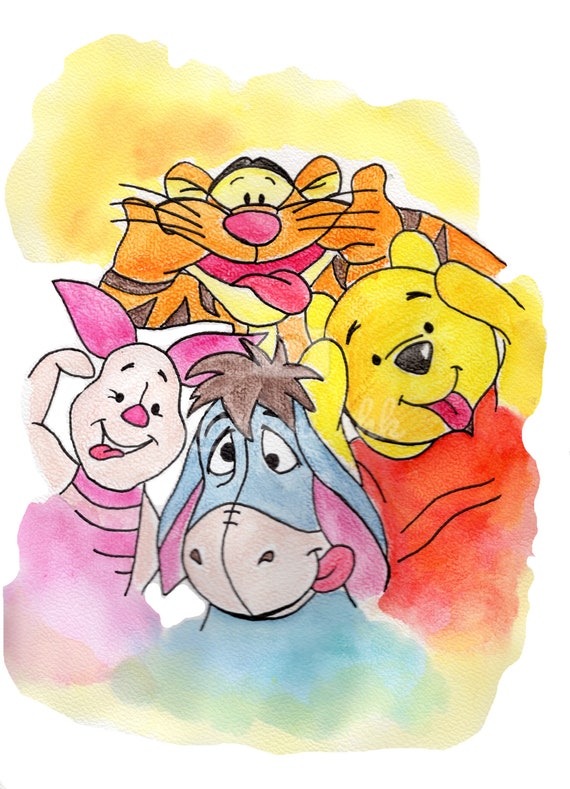This handcrafted watercolor illustration of Winnie the Pooh characters is set against a vibrant background with hues of yellow, pink, and blue seamlessly merging into the characters’ colors. Positioned in the image are Tigger at the top, Piglet on the bottom left, Eeyore in the bottom center, and Winnie the Pooh on the right. Tigger, with his iconic orange and stripes, is tucked behind the others. Piglet, clad in his pink-striped shirt, appears on the left. Eeyore, in shades of blue, has his red tongue showing and brown hair accentuated. Winnie the Pooh on the right dons his classic red shirt, all with their tongues playfully sticking out, giving the sense they are posing for a whimsical photo. The upper bodies are delicately detailed, likely using pencils and coloring pens, while the lower portions blur into abstract watercolor washes, melding the characters into their colorful backdrop.